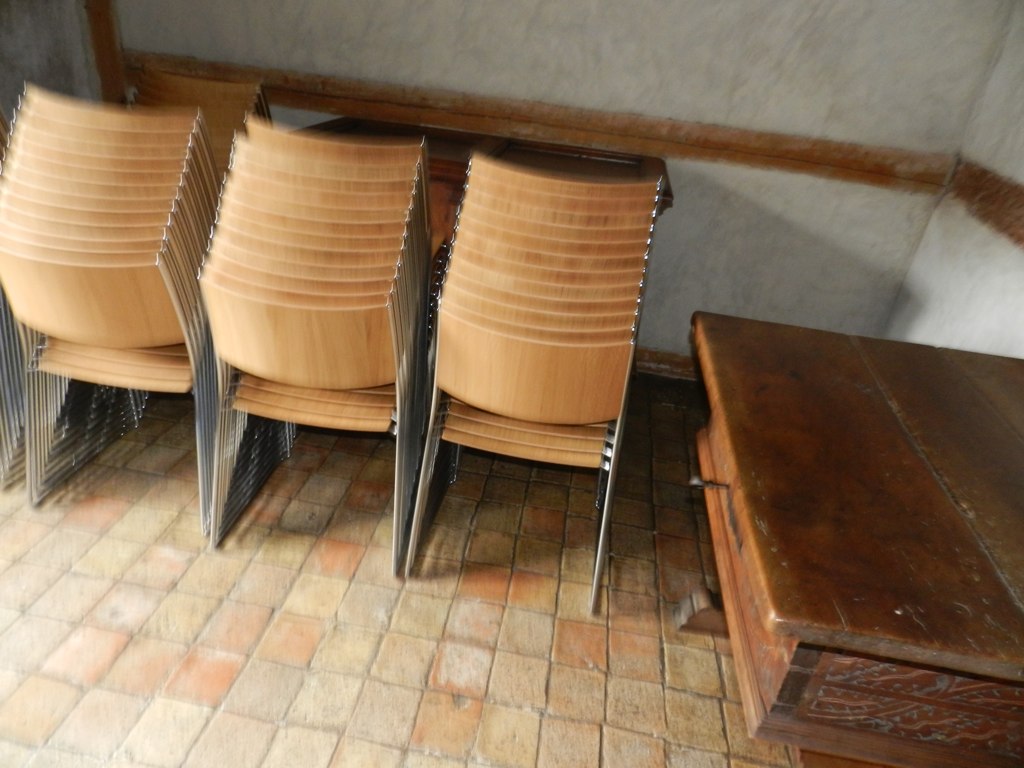The photograph captures a room with notable motion blur, suggesting the camera was in motion when the image was taken. The floor consists of small, square tiles arranged in rows, resembling outdoor bricks in an orange and tan color scheme, and appears scuffed and worn. Dominating the center of the room are three tall stacks of hard conference chairs, each stack containing twelve brown chairs with wooden-looking backs and seats supported by silver metal frames. In the right-hand side of the image, a heavy, dark brown wooden table stands with a design on its side that resembles tiles. A black key protrudes from a drawer in the table. Against the walls behind and to the right of these chairs, the room has a wooden border mid-wall, grayish-white or stone-colored walls, and brown trim at the bottom. There is an indistinct detail in the corner that could be a spider web, adding to the worn and aged atmosphere of the room.